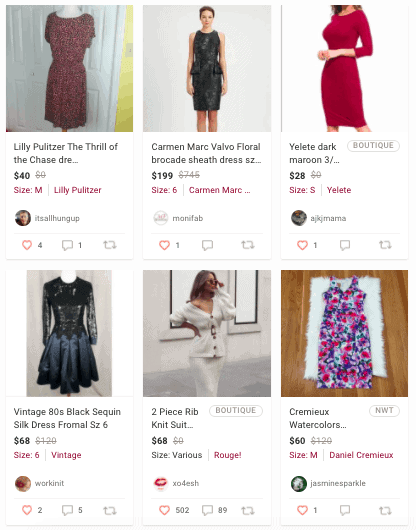The image showcases a meticulously organized online shopping interface for women's clothing. There are six distinct sections, each displaying a different item with detailed information beneath each visual representation.

- In the first section, at the top, is a "Lily Pulitzer The Thrill of the Chase Dress" priced at $40, available in size Medium. It is indicated to be a Lily Pulitzer item and has garnered four hearts and one comment.
  
- Adjacent to it is a "Carmen Mark Valvo Floral Brocade Sheath Dress," available in size 6 and priced significantly higher at $199.

- Moving further, there's a "Yelty Dark Maroon Dress" priced at $28, available in size Small. This item has received one heart and no comments.

- On the bottom row, there's a "Vintage 80s Black Sequin Silk Dress," listed for $68, available in size 6. It's worth noting that there is a typographical error where 'formal' is misspelled as 'fromal.'

- Next, there's a "Two-Piece Rib Knit Suit," though specific pricing and size details are not mentioned in the voice caption.

- Lastly, the "Cremeux Watercolors Dress" is shown, priced at $60 and available in size Medium.

The image captures a variety of dresses ranging from vintage to contemporary styles, providing shoppers with detailed options for different preferences and budgets.